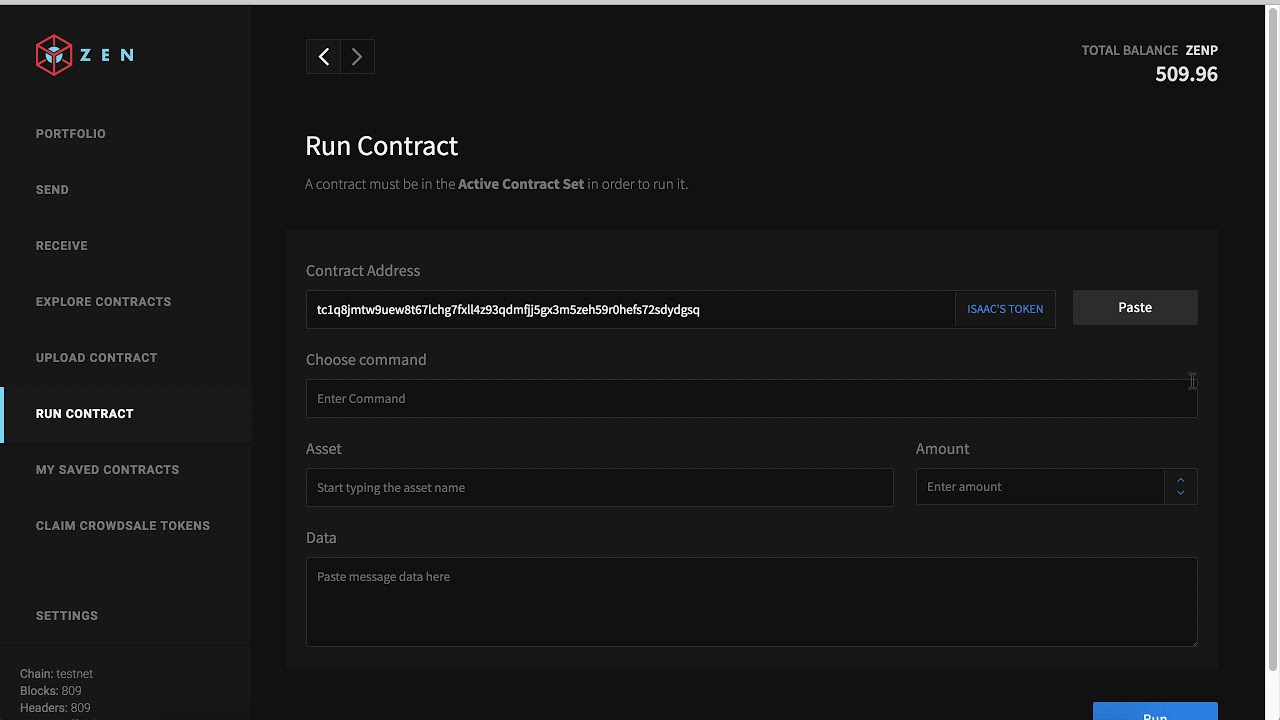**Detailed Caption:**

This image showcases a user interface of a blockchain or cryptocurrency platform named "Zen". Prominently featured in the center is a red cube logo alongside the name "Zen." Below the logo, a structured menu displays various options: "Portfolio," "Send," "Receive," "Explore Contracts," "Upload Contract," "Run Contract," "MySafe Contracts," "Claim," "Casual Tokens," and "Settings."

To the sides, there are navigational arrows indicating "left arrow" and "right arrow" functionality. In the user account section, the "Total Balance" is displayed prominently as "ZENP 509.96."

The "Run Contract" section includes a detailed message stating that a contract must be in the active contract set to be executed. It lists fields such as "Contract Address" beneath the instruction, followed by fields for entering token details ("I have a huge token" displayed in white text), a paste button, and command options. 

Further detailed fields include "Enter Command," "Asset," where users must type in the asset name, "Amount" for entering the transaction amount, and "Data," for pasting message data. The interface also has a gray square element in the bottom right corner which is blue, contrasting against a gray backup. The image is visually dense with text and resembles a typical cryptocurrency or blockchain management interface.

This detailed arrangement suggests it is a comprehensive and professional platform for managing various blockchain and cryptocurrency transactions and contracts.